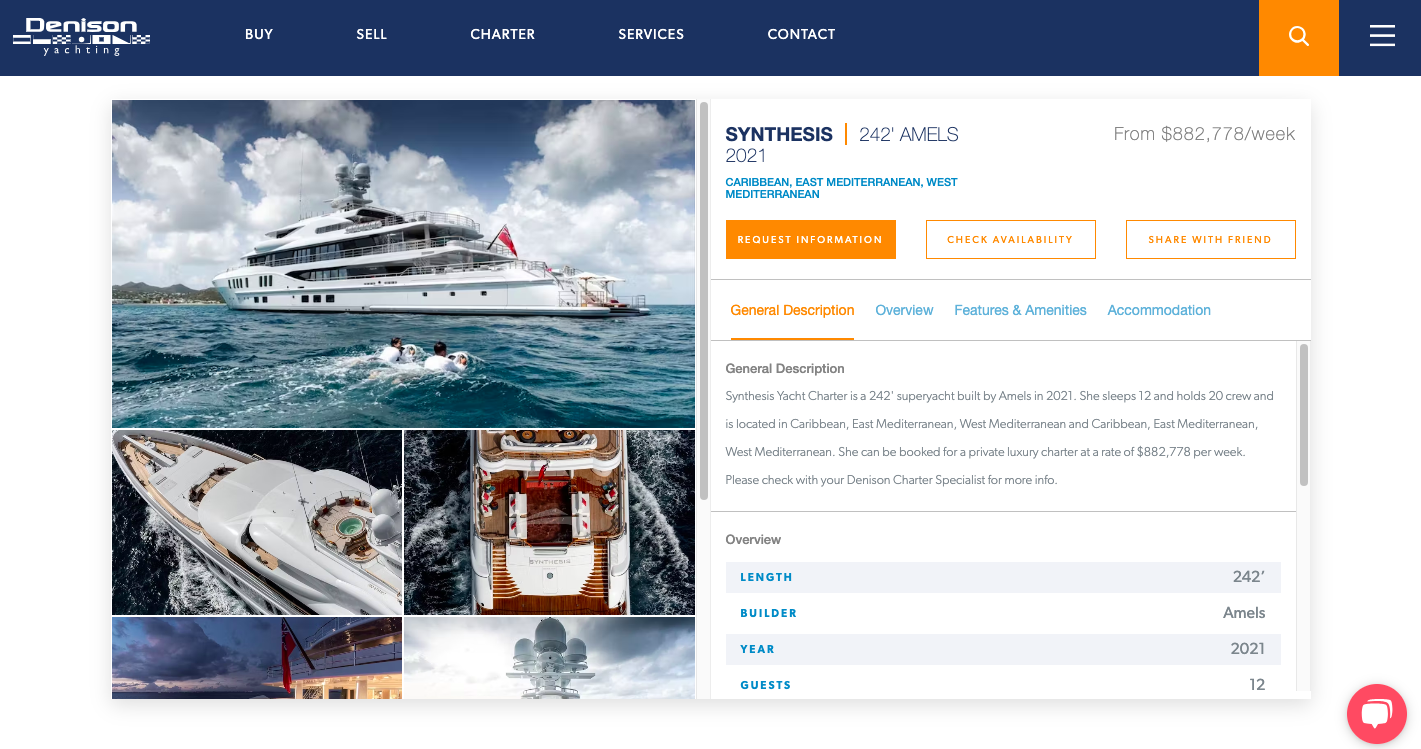In this screenshot from the Denison Yachting website, the upper left corner features a blue banner displaying the company's name in white text: "Denison Yachting." Adjacent to the company name, the banner lists navigation options: "Buy," "Sell," "Charter," "Services," and "Contact."

Below the banner, on the left side of the screenshot, are five vibrant color photographs. The top image captures a stunning white yacht gliding over serene blue waters. The lower left image presents an aerial view of what appears to be a fishing boat. Adjacent to this, another aerial shot showcases a different boat from above.

To the right of these images, detailed information about a particular yacht is displayed: "Synthesis 242 mls 2021 from 882,778 for the week." Below this text, there are three highlighted options within orange-bordered boxes: "Request Information," "Check Availability," and "Share with Friend."

At the bottom of this section, general descriptive categories are listed. In orange text, headings such as "Overview," "Features and Amenities," and "Accommodation" are clearly defined, followed by further descriptive text in blue.